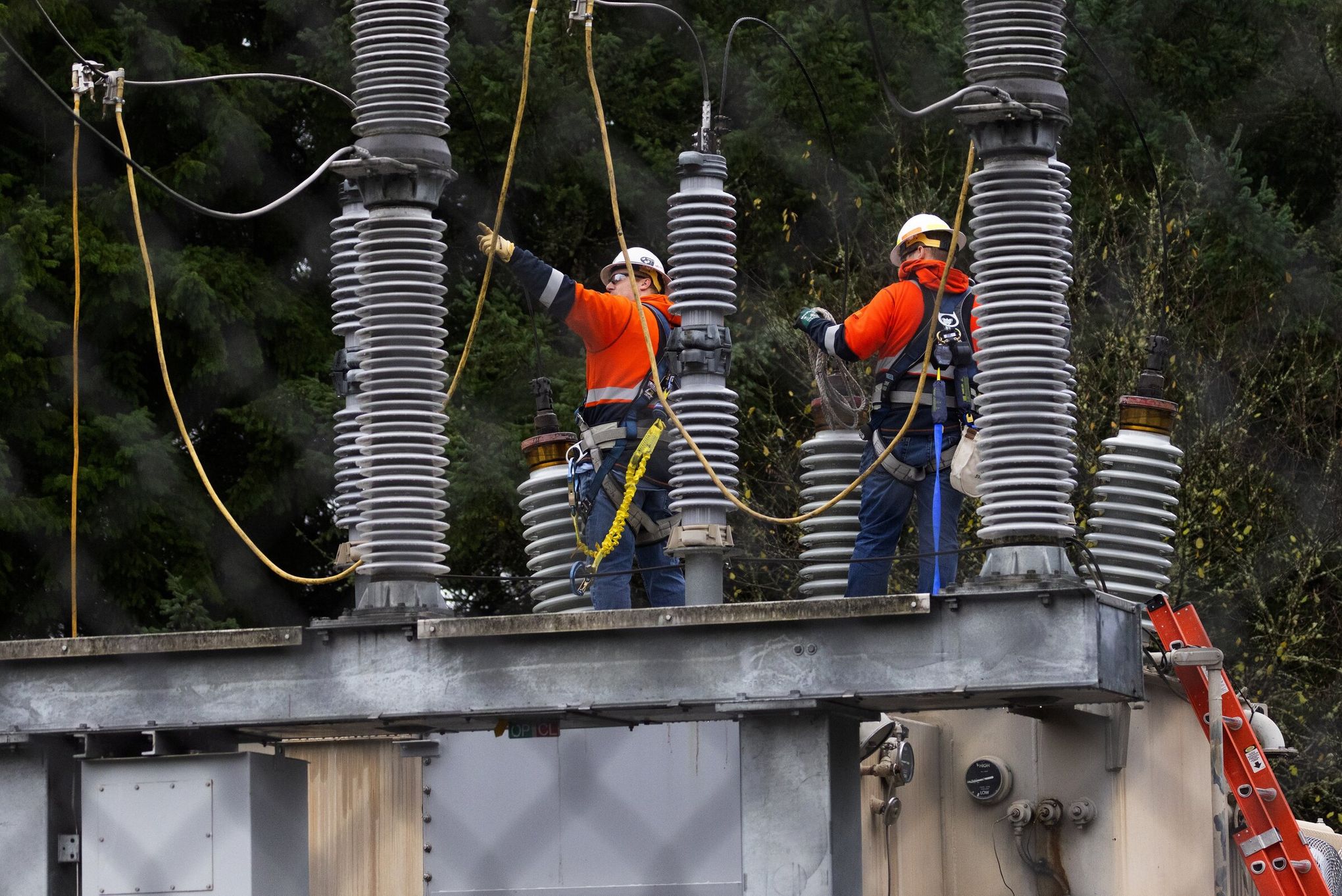In this detailed image, two electricians are working on an elevated electrical transformer within an outdoor substation, surrounded by a thick forest of pine and deciduous trees. Both men are dressed in orange jackets with reflective striping, white hard hats, and blue jeans, complemented by utility belts and black safety harnesses that secure them to the platform. They are standing on a metallic surface that features numerous dials, tubes, and six pylons wrapped in wire or metal detailing. An orange ladder leans against this surface, extending from the ground below to the platform. The man on the left, wearing tan gloves, is pointing towards the upper left corner of the image, while the man on the right, in black gloves, holds an object he is examining. In the background, a bush with yellow leaves or blooms adds a touch of color, contrasting with the dense greenery.